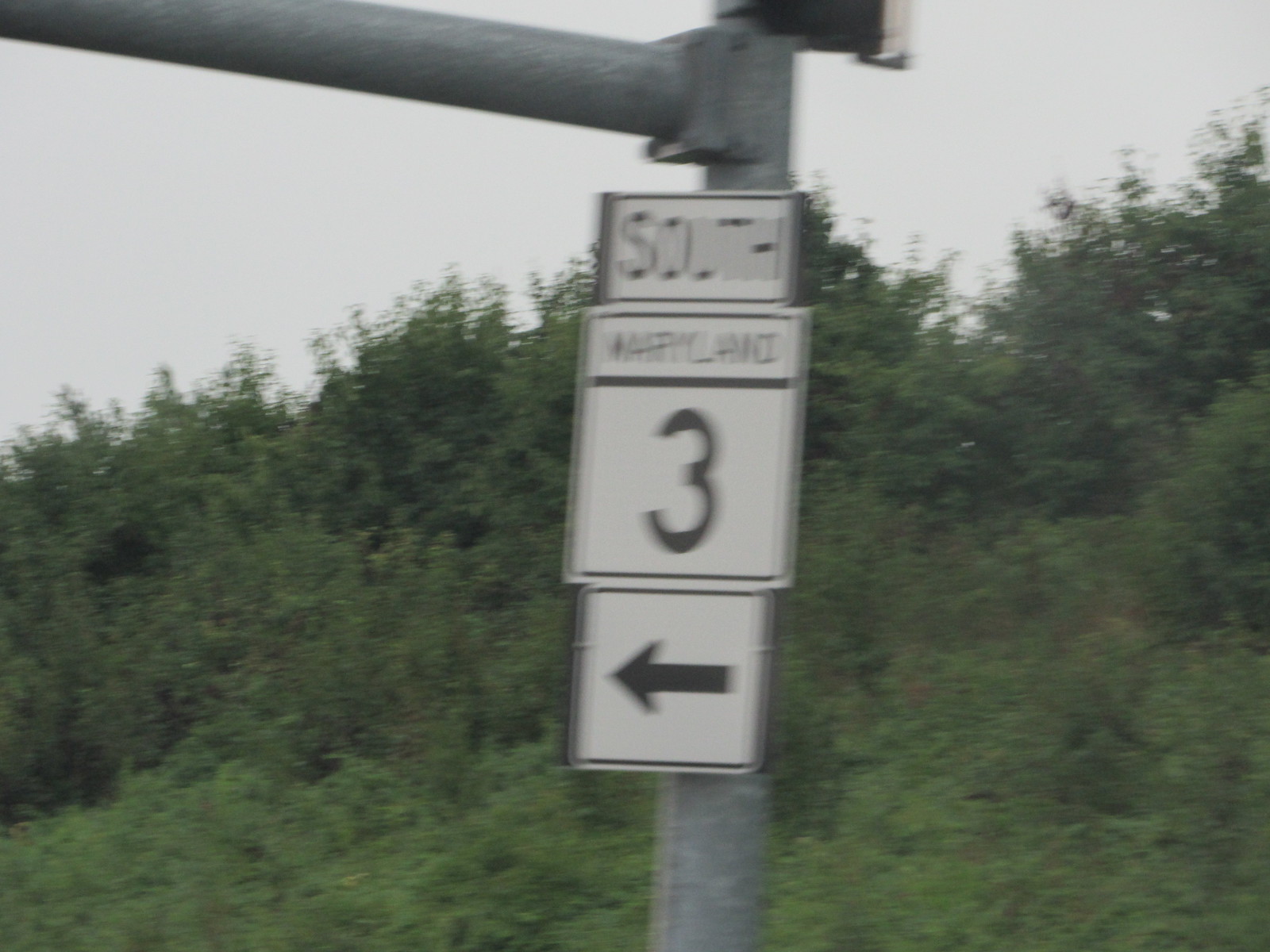This photograph, though slightly blurry, prominently features a street sign mounted on a silver pole. The sign has a white background with the word "South" clearly printed at the top in black font, followed by additional text that is too blurry to decipher. Below the text, a black line separates it from a large black number "3" and an arrow pointing in a direction. In the background, lush green trees and dense foliage are visible, hinting at a natural, perhaps suburban, setting. The sky is overcast, evidenced by a gray hue. Above the sign, the top of another metal pole is partially visible. Despite the image's graininess, the scene is rich with detail.